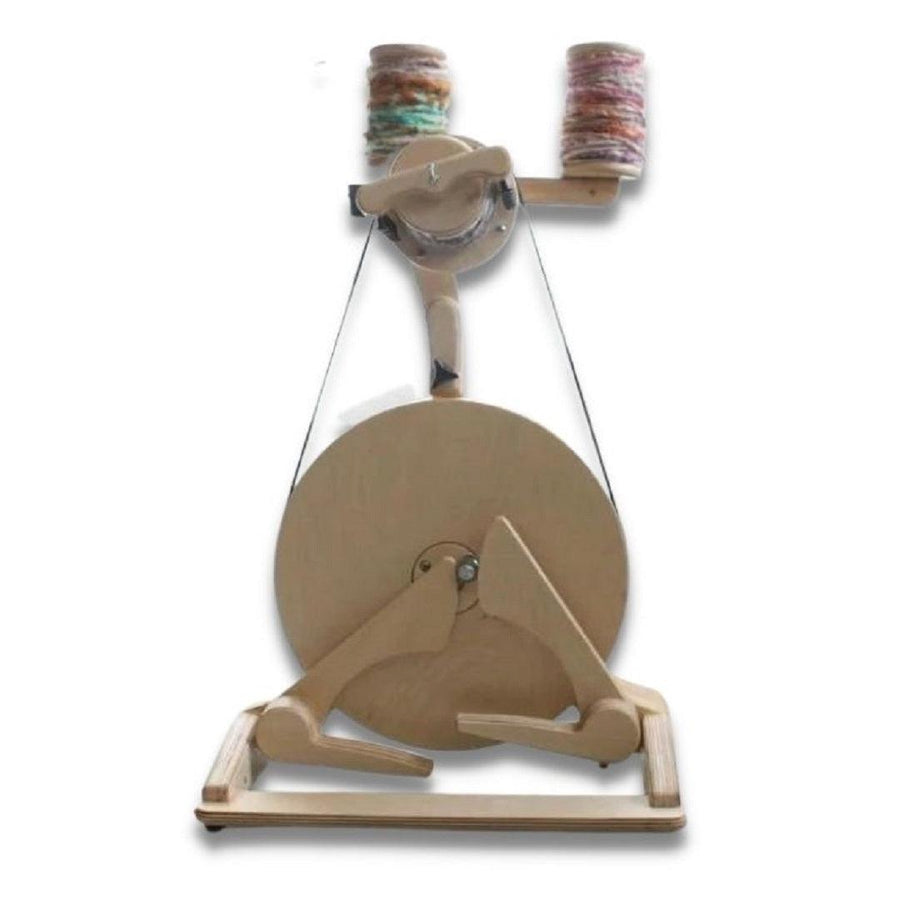The image captures a detailed view of a vintage, manually-operated yarn winder, primarily crafted from wood with some metal components. At the top of this intricate machine, there are two spools of yarn, each featuring a colorful array of threads in shades of magenta, orange, teal, brown, pink, and white. The yarn from these spools is threaded through a smaller circular mechanism positioned just below them, which then connects to a larger, record-like disc at the base of the machine. 

This larger disc appears to function as a main winding area, supported by a robust wooden base that ensures stability. The machine also includes two extending arms on either side, likely aiding in the winding process, though their exact function is not entirely clear. The yarn winds down from the smaller upper circle to the more substantial lower disc, suggesting a transfer and organizing mechanism. The backdrop of the photograph is a neutral white with some subtle shading, which helps to focus attention on the intricate details and craftsmanship of the yarn winding device.